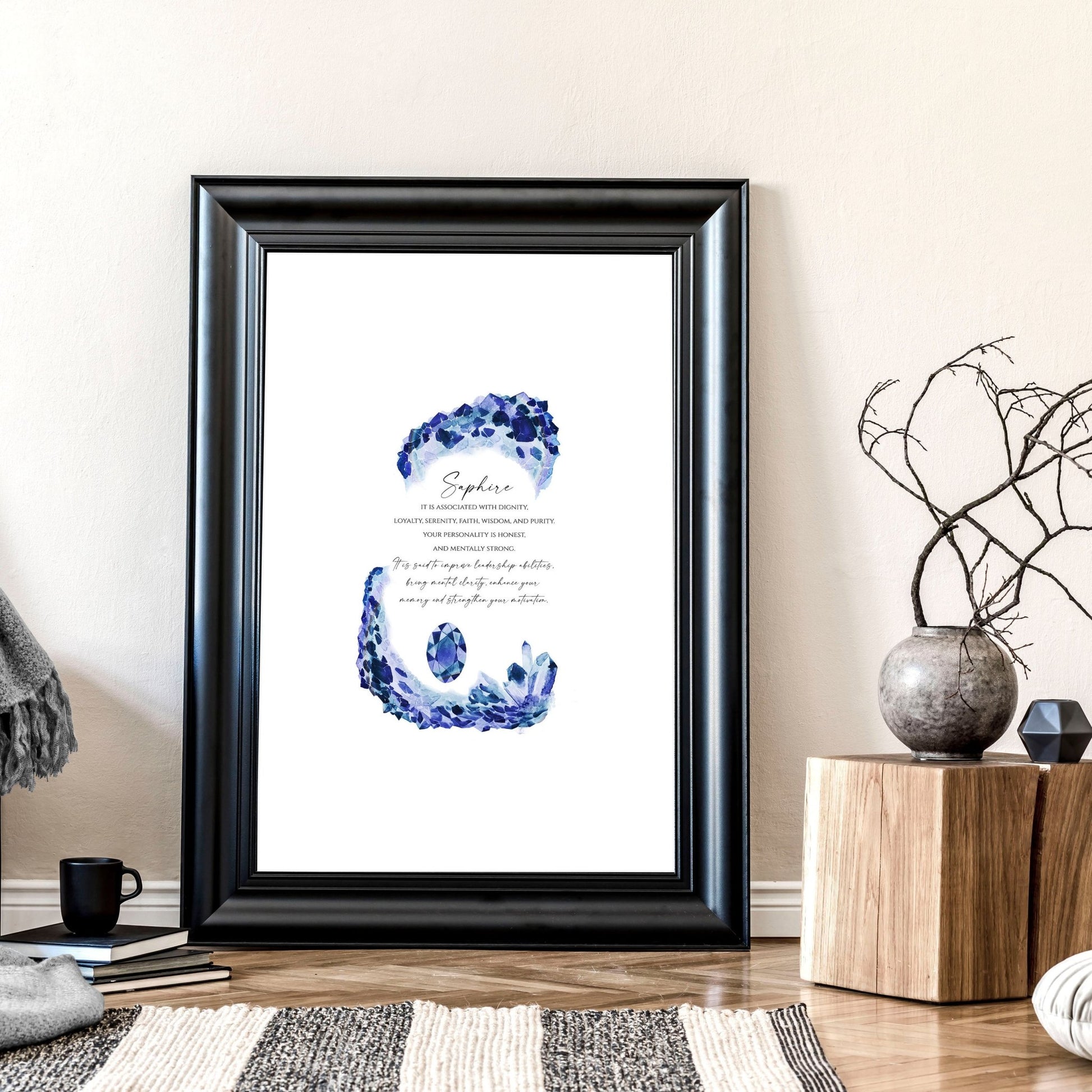The image showcases a meticulously arranged interior scene, focused on a framed artwork leaning against a white wall with white baseboards. The black matte frame contains a piece of art with a central blue crystal and the word "Sapphire" prominently displayed. Below the title, the text elaborates on the attributes associated with sapphire, such as dignity, loyalty, serenity, faith, wisdom, and purity, although the bottom part of the text is slightly blurry and difficult to read. The frame is positioned on a wooden floor, partially covered by a black and white striped area rug.

To the right of the frame, a plush pillow is visible on the floor. On the left side, there is a stack of three books topped with a black coffee mug. Adjacent to this is a wooden block featuring two objects: a gray vase with bare tree branches protruding from it and a small, geometric black sculpture resembling a star. Out of the image's immediate frame, there seems to be a throw or blanket hinted at. The overall composition is minimalistic and cozy, blending natural elements with artistic touches.